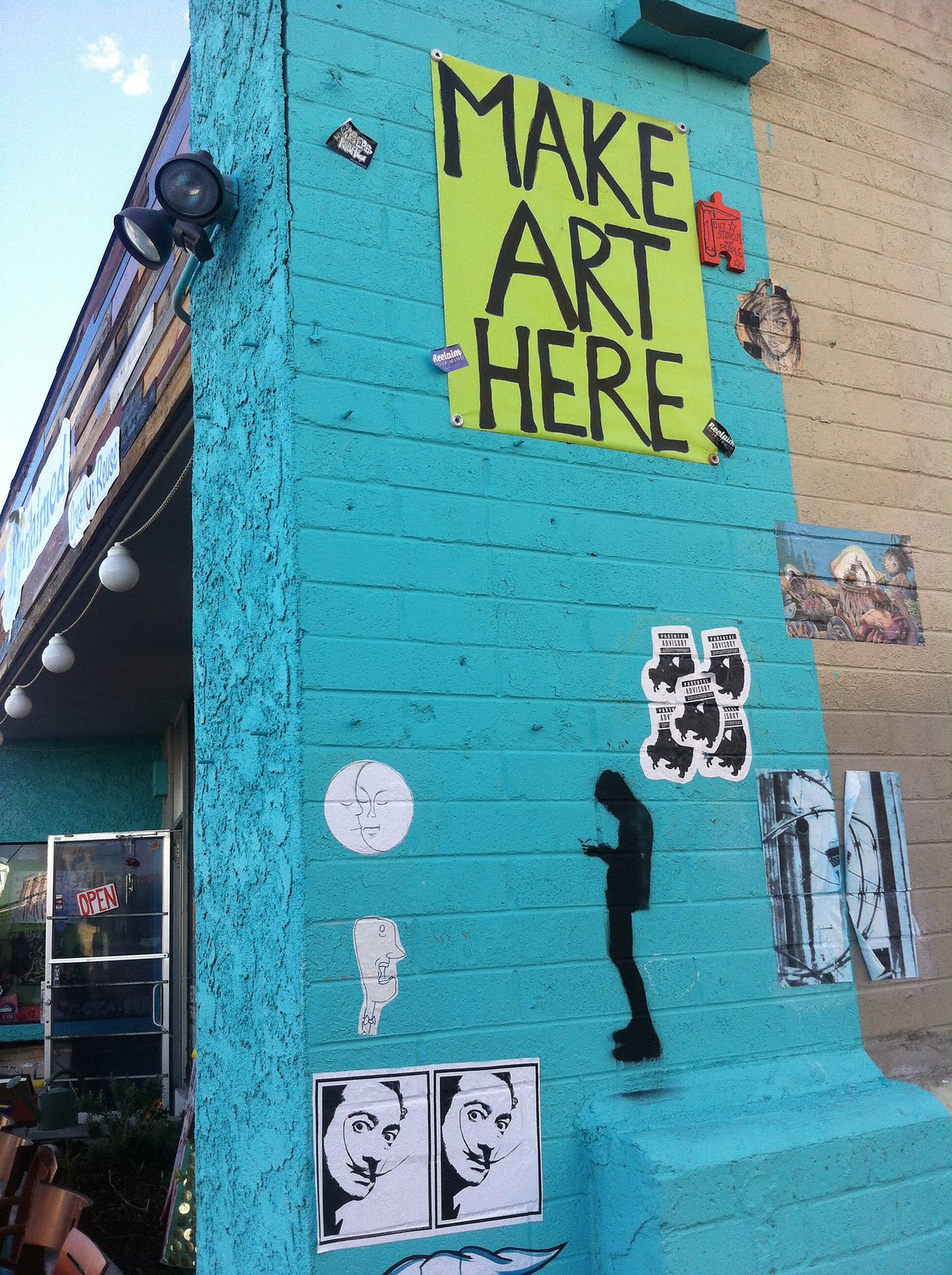The photograph captures the sidewall of a brick building adorned with various artworks and stickers on a clear day with a few clouds in the light blue sky. The brick wall features a vivid display of colors, including teal, black, white, blue, red, orange, gray, copper, brown, green, and others. A yellow cardboard sign with the text "MAKE ART HERE" in bold black marker is prominently displayed on the blue-streaked section of the wall. The building also has a silhouette of a person leaning back and looking at something in their hands, among other drawn pictures such as a monkey, a man with a long mustache, animals, and barbed wire. The setting includes a middle door labeled "OPEN" and flood lights at the top of the building, as well as multiple signs and some buckets positioned out front.